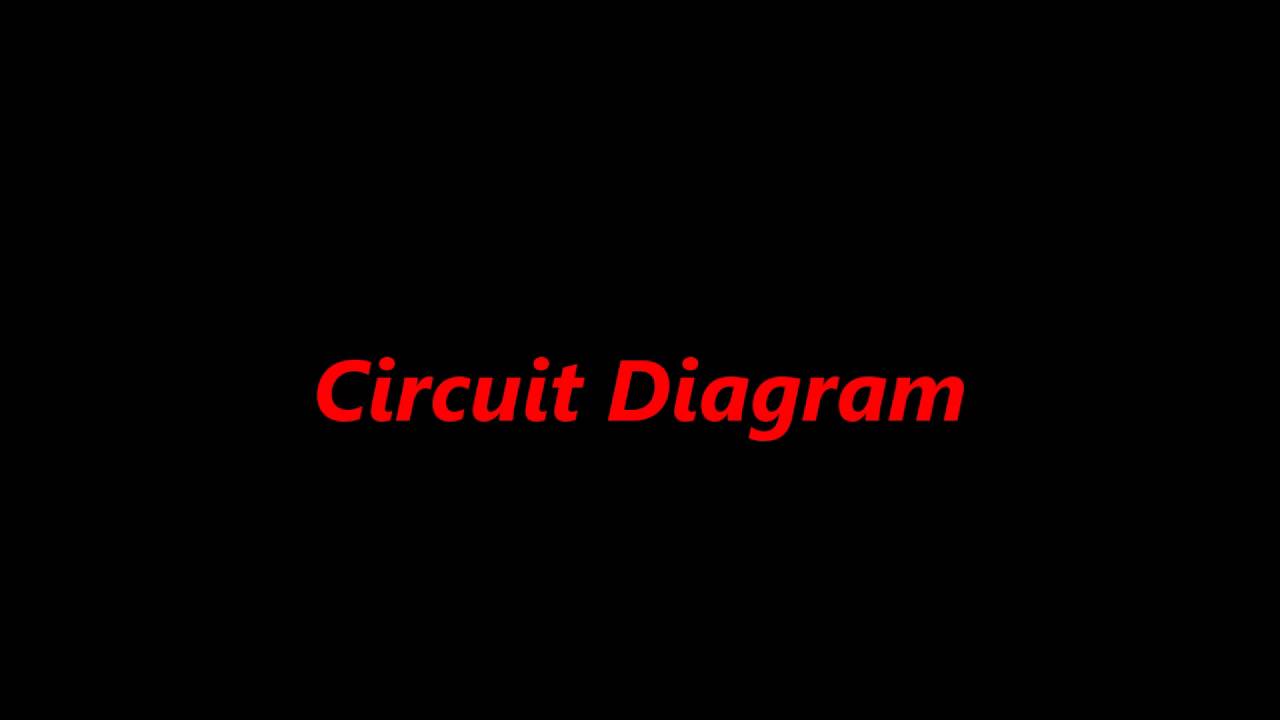This image features a text-based layout with a minimalist design, primarily dominated by the words "Circuit Diagram." The background is a solid black, serving to highlight the text, which is rendered in striking red italics. Positioned centrally, slightly towards the bottom of the rectangular, horizontally oriented frame, the words stand out crisply against the dark backdrop. The overall composition suggests it might serve as a title card or an introductory slide in a presentation, possibly used on a website to capture attention before viewers engage with more detailed content, such as a PDF. The absence of any additional graphics or elements emphasizes its simplicity and straightforwardness.